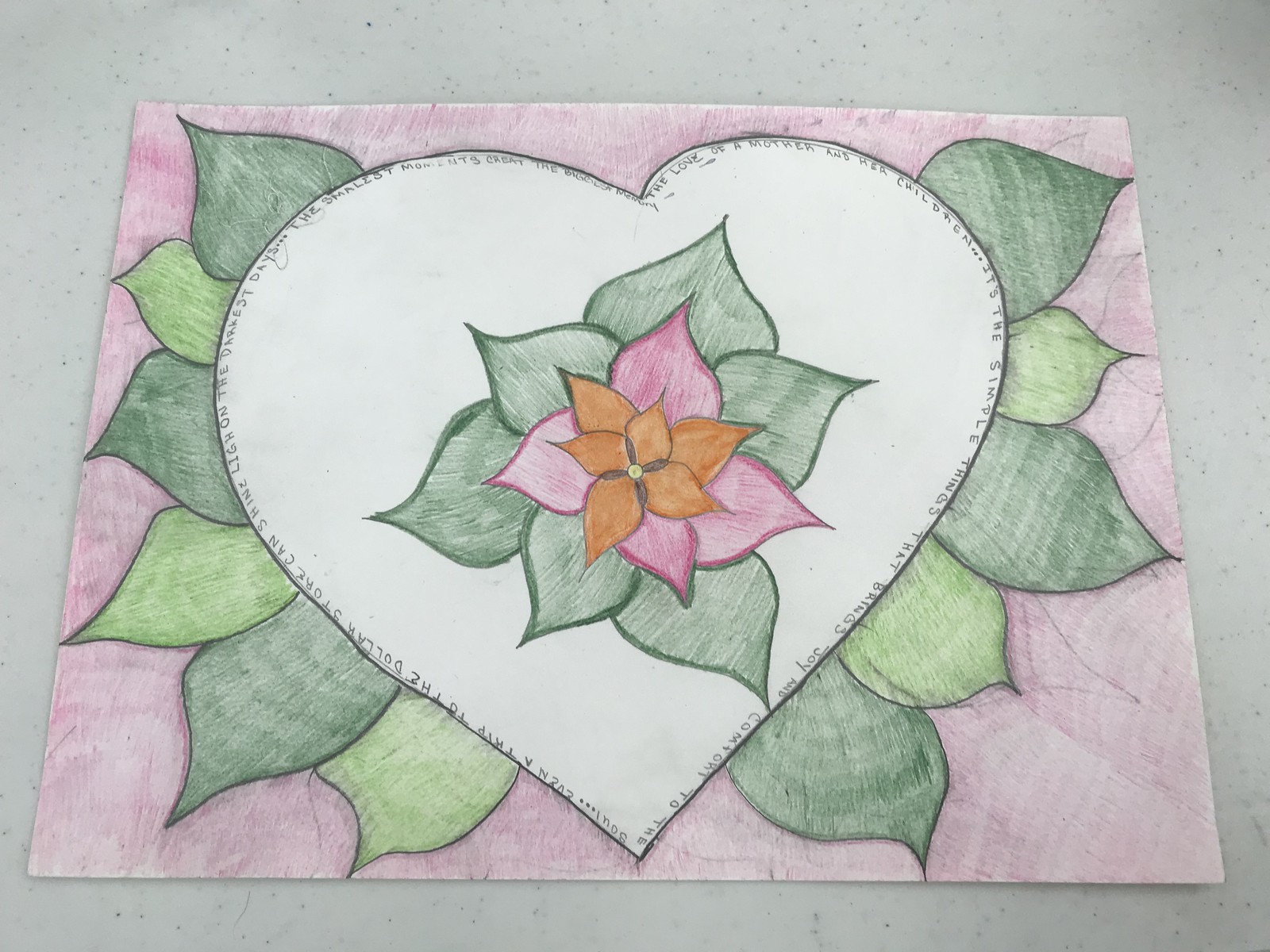The image depicts a hand-drawn sketch on a rectangular piece of paper placed on a white marble countertop speckled with tiny black dots. The paper has been colored pink, especially around the edges, using crayon or colored pencil. At the center of the drawing is a large heart outlined in black with its interior mostly left white. Surrounding the heart are alternating dark green and light green leaves, some of which are slightly smaller than others but generally similar in shape and size. Within the heart, there's a sequence of leaves that get progressively smaller toward the center: starting with the largest, which are dark green, then transitioning to pink, and culminating in a flower-like structure with four orange petals and a yellow center. The border of the heart is adorned with finely written text in black ink, containing phrases such as "the love of a mother for her children" and "it's the simple things that bring joy." The text follows the curvature of the heart and appears to include various other sayings, though some of it is hard to read, and segments are upside down.